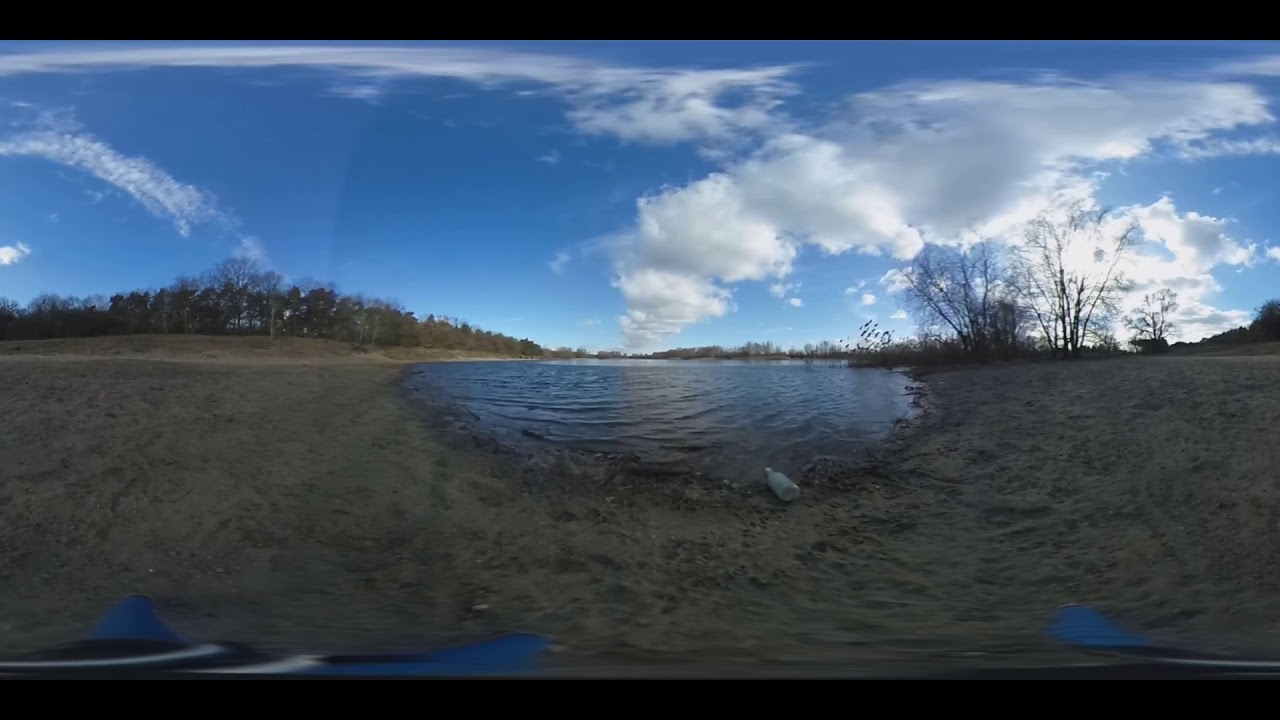In this panoramic outdoor shot, the top half of the image is dominated by a vast, clear blue sky with scattered cumulus and nebulous clouds, which curve slightly due to the wide-angle photography. Below the sky, the center of the image prominently features a shallow body of water, possibly a pond or large puddle, surrounded by dirt. The water appears murky and calm, with an old plastic bottle discarded near its shoreline, suggesting some littering. On the left side of the water, there are green trees, while the right side has more trees and plants, some of which are barren and reduced to sticks. The surrounding area is natural, populated with trees and brush. In the foreground, dirt and a few scattered plants frame the scene. The sun is low in the sky, either setting or rising, casting a gentle light that illuminates the clouds and the landscape, adding depth and perspective to the image. Overall, it's a serene yet slightly neglected natural setting, with a flock of ducks visible, possibly about to take flight into the expansive blue sky.